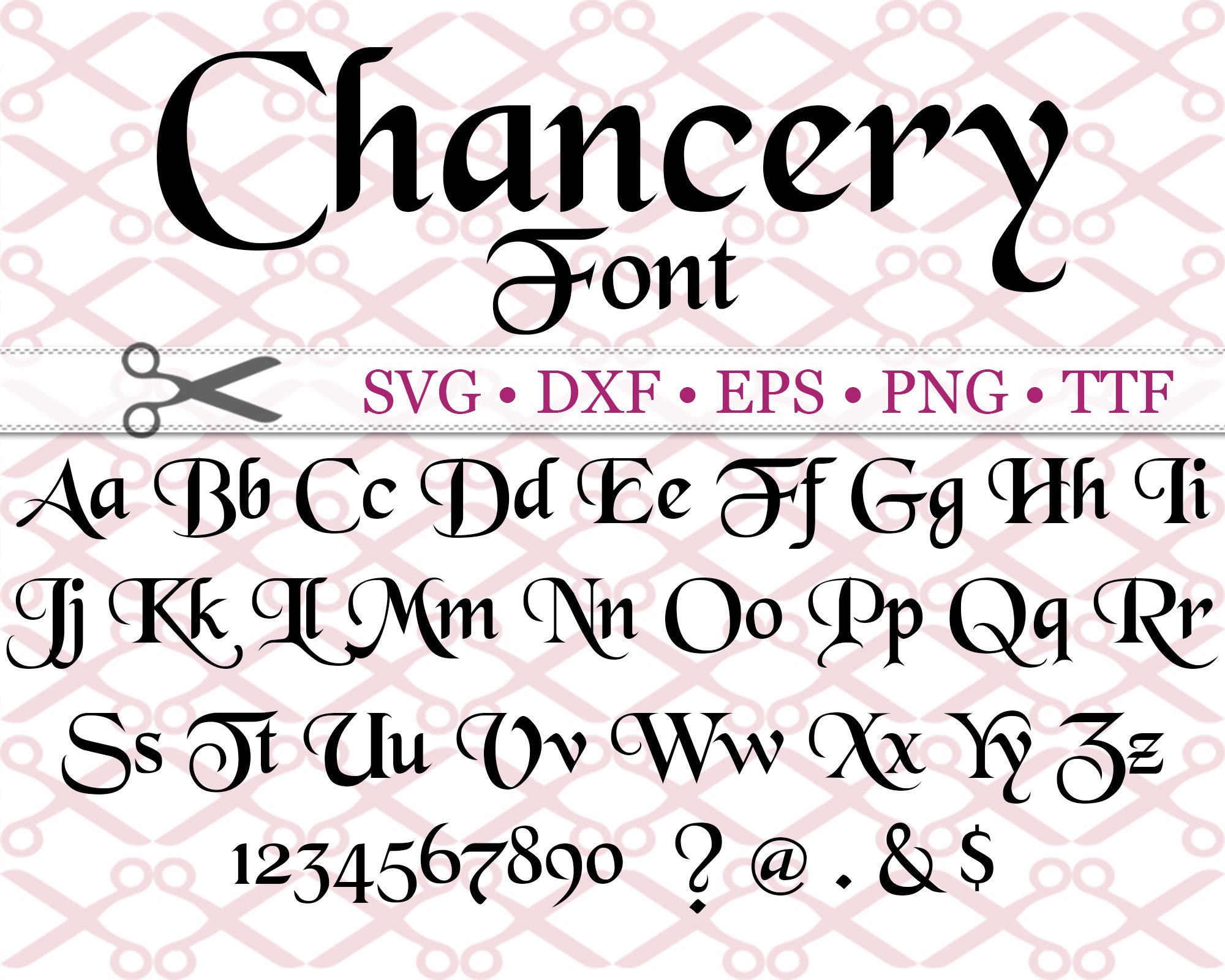The image is a rectangular banner displaying a font titled "Chancery." The background is white with a repeating pattern of pink scissors. At the top, in large black text, it reads "Chancery Font" in Chancery script. Directly beneath this, a ribbon-styled banner spans the width of the image and contains purple text listing available file formats: SVG, DXF, EPS, PNG, and TTF. Below the ribbon, there are four rows showcasing the Chancery font: three rows of both uppercase and lowercase alphabets (e.g., AA, BB, through to ZZ), and a fourth row showing numbers (0-9) and special characters (e.g., question marks and other symbols). On the right side, a gray pair of scissors is depicted. The overall layout and repeated motifs emphasize the versatility and elegance of the Chancery font.